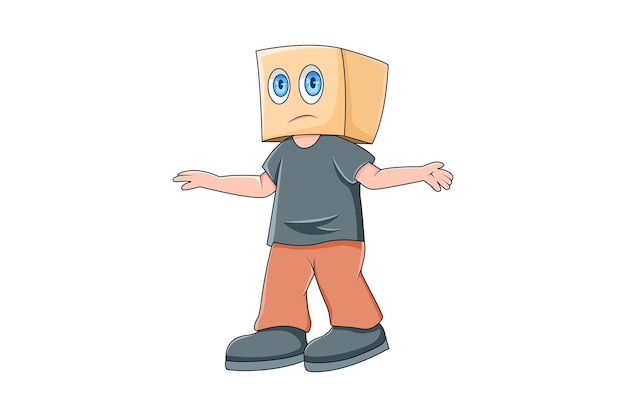The illustration features a cartoon character against a stark white background, emphasizing the character. This character sports a cardboard box or possibly a paper bag for a head, which is brown and square-shaped. The head has blue eyes with black pupils set against white backgrounds, and a frowning mouth depicted as a single line. The character’s body is human-like, with white skin visible on the arms and upper chest or neck, and the arms are extended outwards from the torso. The character is dressed in a gray or blue shirt, red or orange pants, and gray or blue shoes. The character is oriented to face the left side of the image, with the back facing right. The overall style is traditional cartoon.